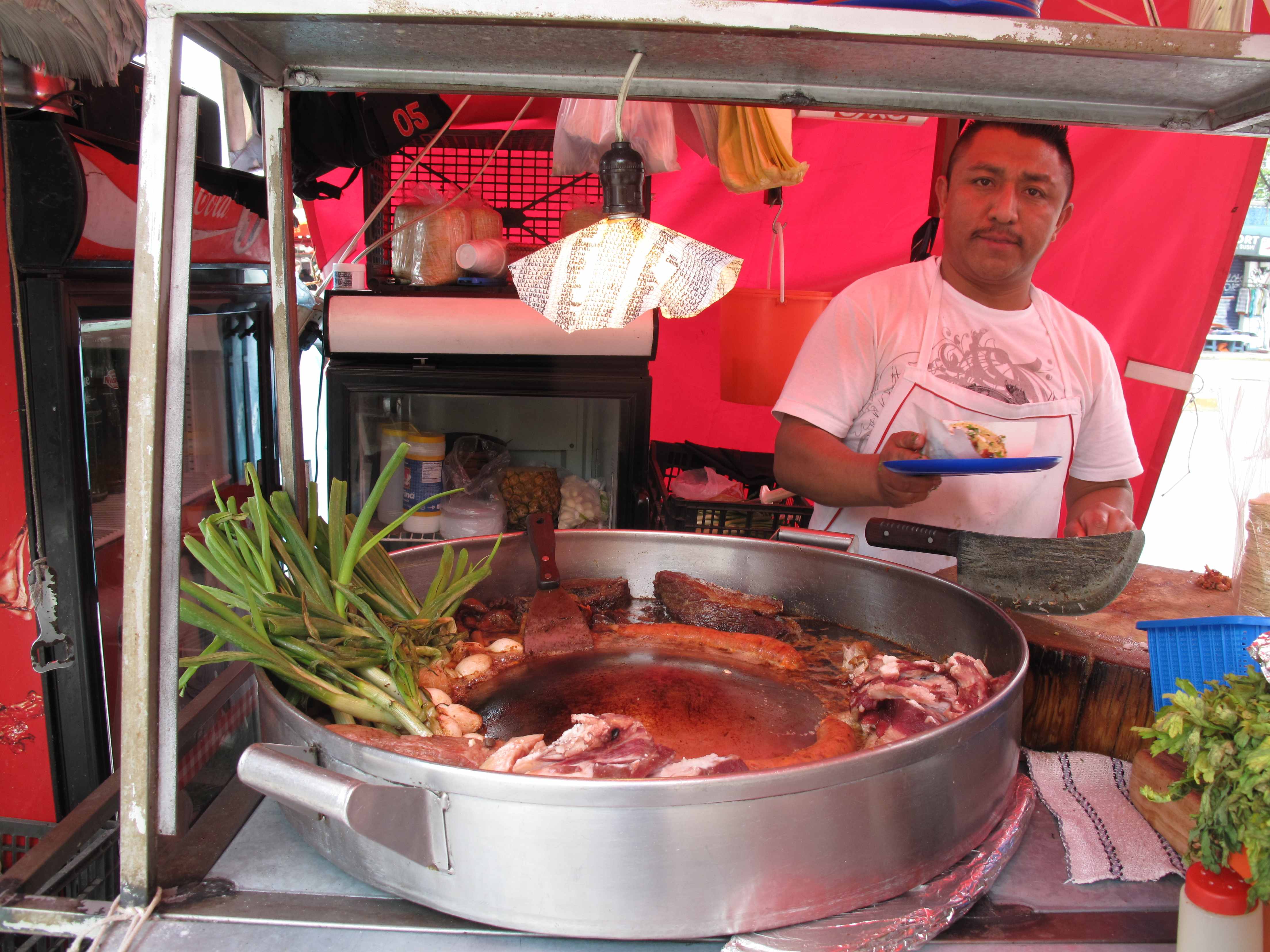In this vibrant image set in an outdoor market, a man of Hispanic or indigenous descent stands at his food cart, which is adorned with a variety of cooking tools and ingredients. He wears a white t-shirt and a white apron, and holds a blue plate featuring a dish that looks like tacos. The cart's front counter prominently displays a large silver pot filled with various meats and herbs, including green onions and cilantro. To the left of the man is a Coca-Cola cooler containing drinks, while behind him there is another fridge and a grill or an oven. A huge knife rests on a butcher block, indicating active food preparation. The backdrop features red curtains that partially reveal the street outside, adding to the dynamic setting filled with colors like pink, blue, green, brown, silver, red, and white.